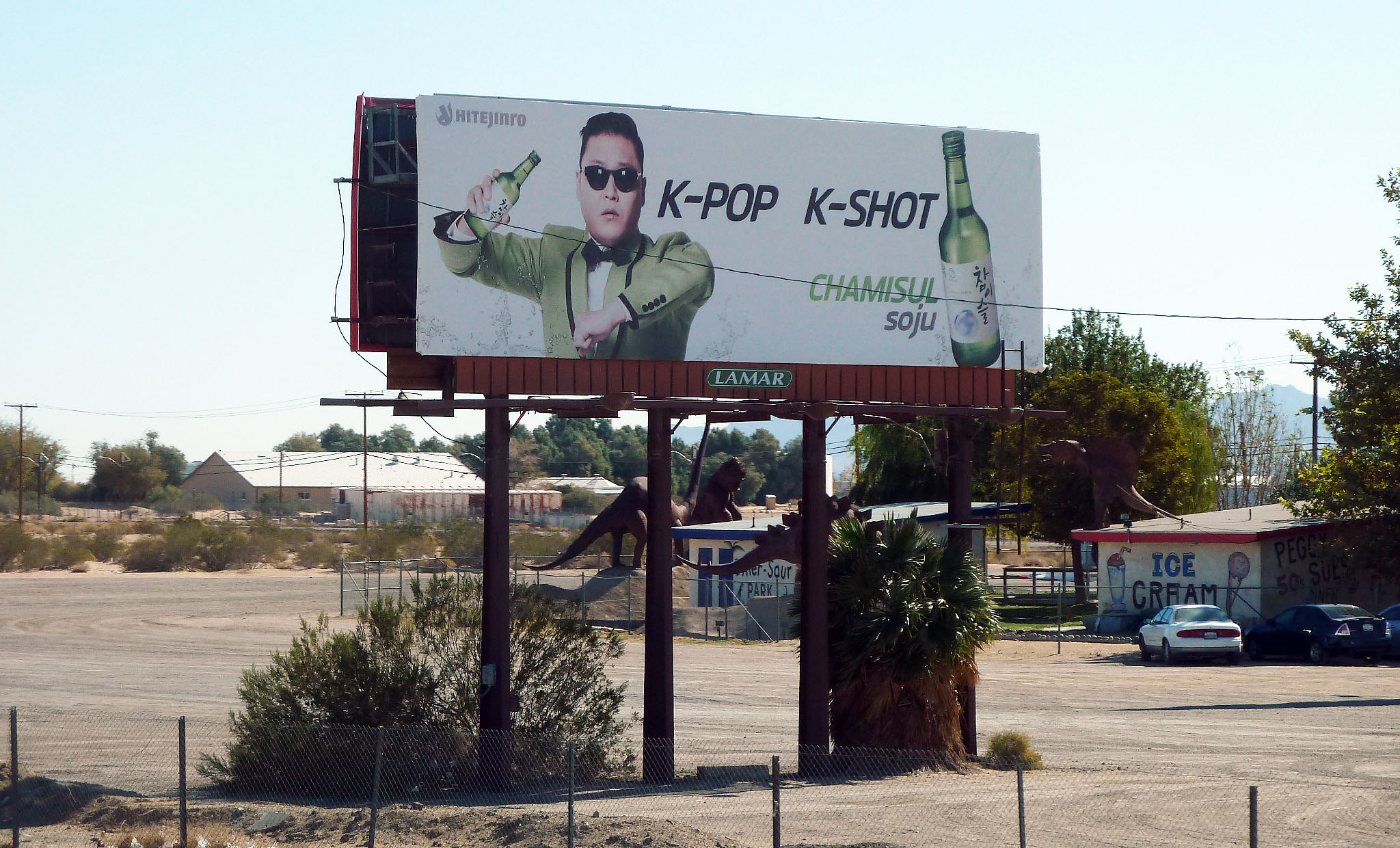The image captures an outdoor scene dominated by a prominent billboard situated on four red metal poles, towering high against a backdrop of a clear blue sky. The billboard features a striking advertisement with a white background, showcasing an Asian man with slicked-back black hair, wearing black, cat-eye sunglasses reminiscent of those worn by Tom Cruise. He is dressed in a distinctive green tuxedo jacket with black trim, a black bow tie, and a white shirt, holding a green bottle with a white label.

The billboard displays the text "K-POP K-SHOT" in bold black lettering on the right side, with "HITE JINRO" in the corner. The green bottle he holds is Chamisul Soju, prominently advertised with the words "CHAMISUL SOJU."

Beneath the billboard, the area is an open, dirt-filled field with a shrubbery bush right below the structure and a house visible on the right-hand side. Surrounding the field are suggestions of a roadside attraction, potentially abandoned, featuring two buildings with fiberglass dinosaur figures and a sign on one building advertising ice cream. A single car is visible, indicating that the location isn't very busy. This scene is set behind a metal fence, lending a somewhat isolated and remote atmosphere to the image.